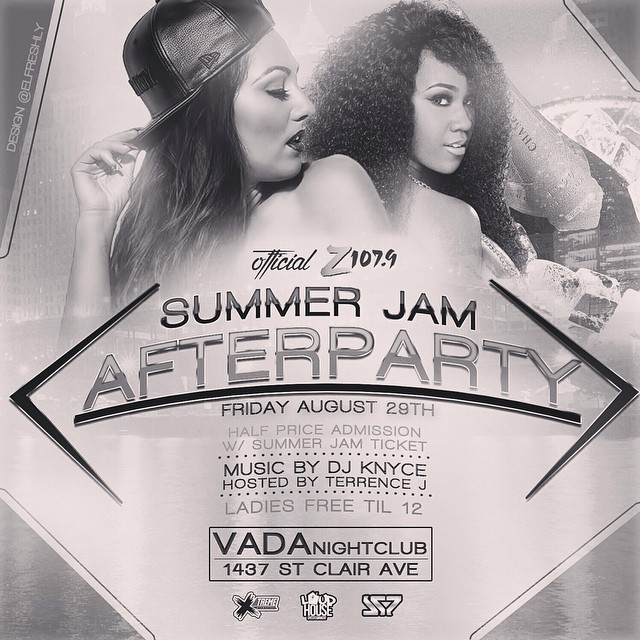This black and white poster advertises the official Z107.9 Summer Jam Afterparty. At the top of the poster are two women. The lady on the left is wearing a backwards leather baseball cap and has long straight hair cascading past her shoulders. She is holding the brim of her cap with her right hand, her fingers bent. The woman on the right has long, curly black hair flowing past her shoulders. She is facing to the right but looks partly forward over her shoulder at the camera, creating an alluring glance. Both of them appear hip-hop styled, adding to the event's vibe. Below the image, large text announces the "Official Z107.9 Summer Jam Afterparty." The event details follow: "Friday, August 29th," "Half-price admission with Summer Jam tickets," "Music by DJ Nice," "Hosted by Terrence J," and "Ladies free till 12." The location is specified as "Vada Nightclub, 1437 St. Clair Avenue." Several icons, including one resembling an upside-down 7, a backwards 7, and another 7, are positioned at the bottom of the poster.